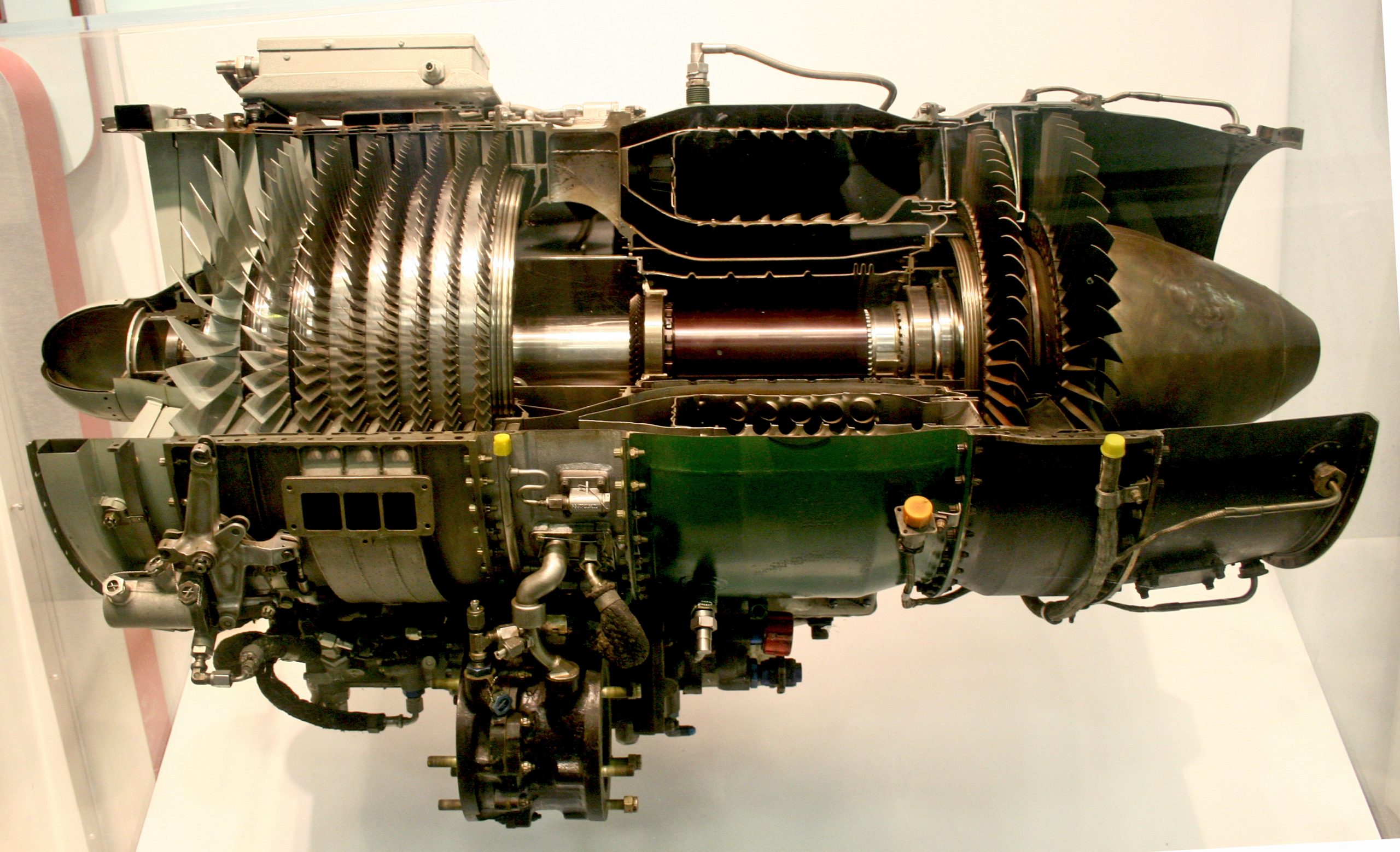This image depicts a complex piece of machinery, likely an airplane or jet engine, extracted from its usual setting and displayed against a white backdrop. The engine is predominantly cylindrical with an uneven, grooved surface, characterized by numerous blades extending from various parts. The structure has a light gray and green shell enclosing internal components and is equipped with multiple fans arranged sequentially. There is a prominent round cylinder in the center, indicative of the rotational mechanism within the engine. One end features a series of fans and a round turning rod, transitioning into a metal-barrier-protected, curved, conical segment, presumably the exhaust system. A conspicuous small cylinder on top is linked by copper wires to a white box, hinting at electrical components vital for the engine's operation. Various tubes and wires interconnect these parts, completing the intricate assembly. The image showcases the detailed, robust engineering typical of high-performance aerodynamic machinery.